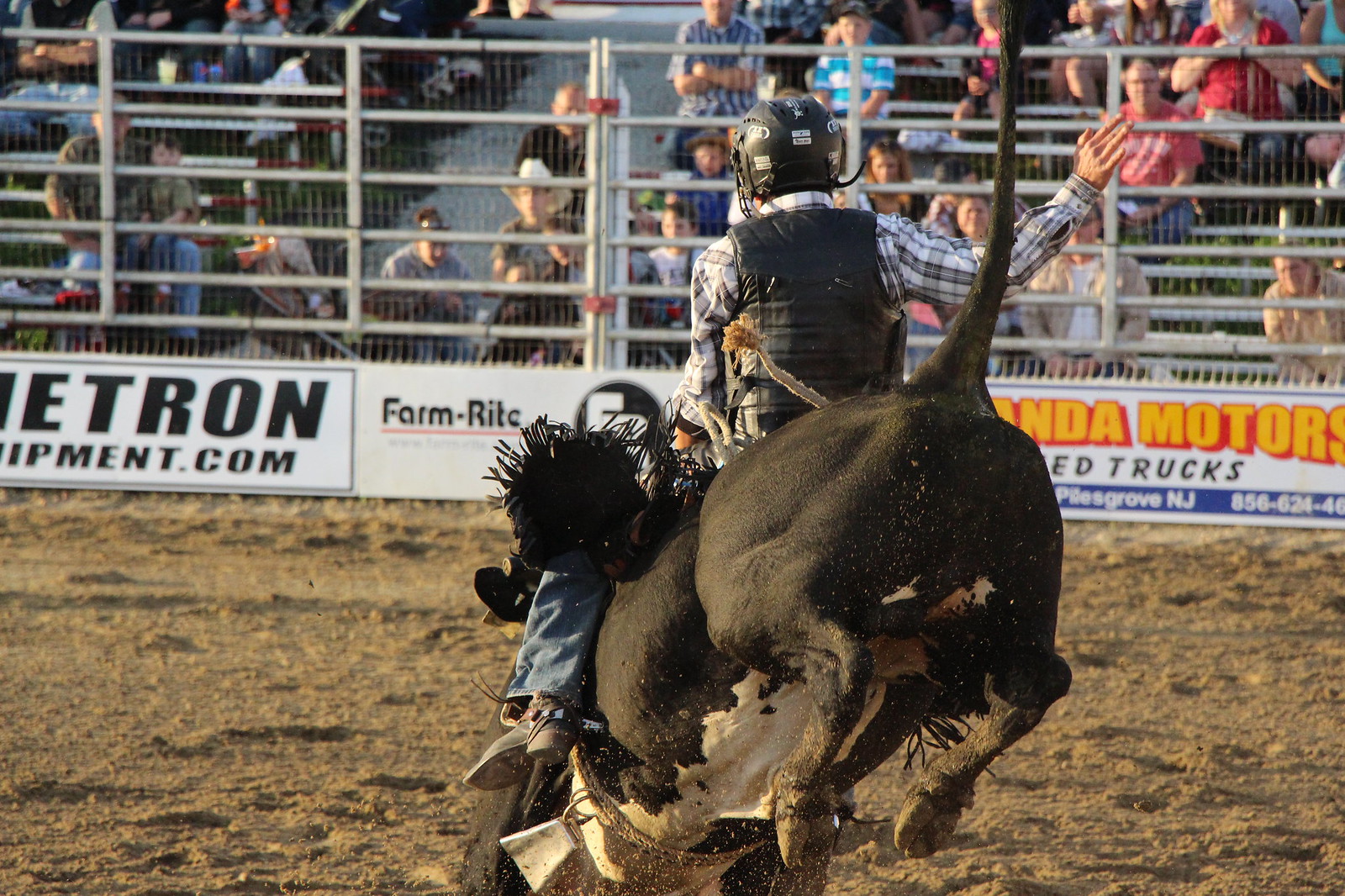This vivid color photograph captures a thrilling moment at a rodeo in landscape orientation. At the center of the dirt-covered ring, a gentleman, donning a black helmet and safety vest, rides a powerful bull. He is attired in a white and black checkered long-sleeve shirt, blue jeans, and cowboy boots. Clinging to the bull with his left hand, the rider skillfully balances his right arm raised high. The dark brown bull, marked with a white belly, is captured mid-rear with its hind legs and tail lifted off the ground, creating a dynamic action shot. In the background, sparse metal stands hold a mixed-gender crowd of spectators, who watch intently. Sponsor banners from companies like Atron, Shipman.com, Farmlite, and others adorn the fence between the arena and the audience, enhancing the authentic atmosphere of this exhilarating rodeo scene.